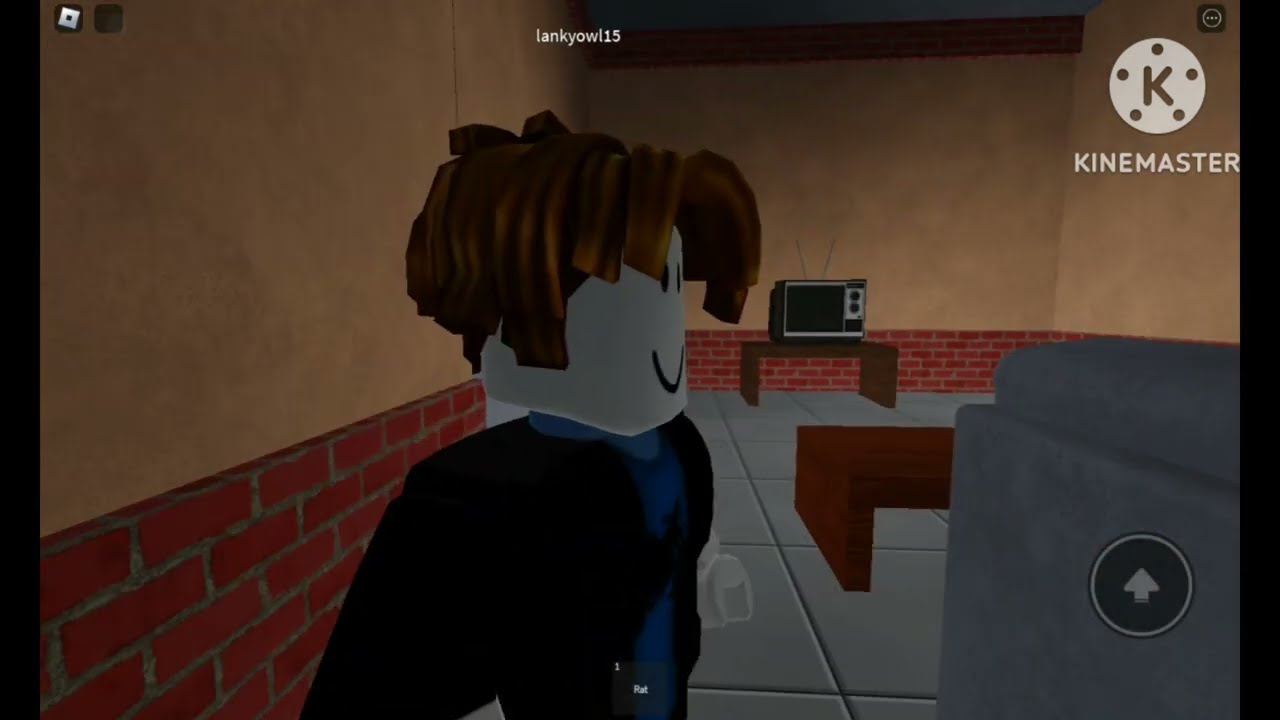The screenshot from the game features a room with a mix of cream-colored and red brick walls. The floor is composed of large gray tiles. In the center of the room stands a Roblox character with short brown hair and a smiling face, dressed in a white and red coat with a blue shirt underneath. The character is facing to the right. The back of the room displays a black traditional TV with antennas, resting on a brown table. Another brown coffee table is located centrally in the room. To the bottom right of the image, there is a gray couch. In the upper middle of the screen, white text reads "LANKYOWL15," while the top right corner features a watermark with "KINE MASTER" inscribed below a white circle containing the letter 'K' and three surrounding dots. The top left corner shows additional on-screen icons.